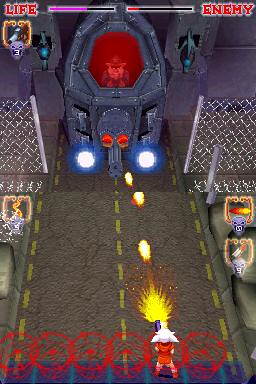The image captures an intense moment of gameplay, showcasing high-stakes action. The scene appears to be extracted from a PC, mobile device, or a TV displaying console gameplay. At the center of the image, a character clad in a vibrant orange outfit is seen wielding a weapon that resembles a bazooka. This character is strategically targeting a formidable, large metallic tank advancing towards them on a road. 

The tank, featuring a conspicuous red shield, partially obscures the view of its pilot, who appears to be a small figure with hands either on a steering wheel or prepared to retaliate. On the left side of the screen, a display indicates the player's life bar at approximately 75%, accompanied by an image or icon representing the character or their weapon. In contrast, the enemy tank's life bar on the right side shows a critically low level, around 15%, suggesting that the tank is on the brink of destruction. This snapshot depicts a climactic battle scenario, emphasizing the imminent victory for the player as they deliver potentially fatal blows to their adversary.